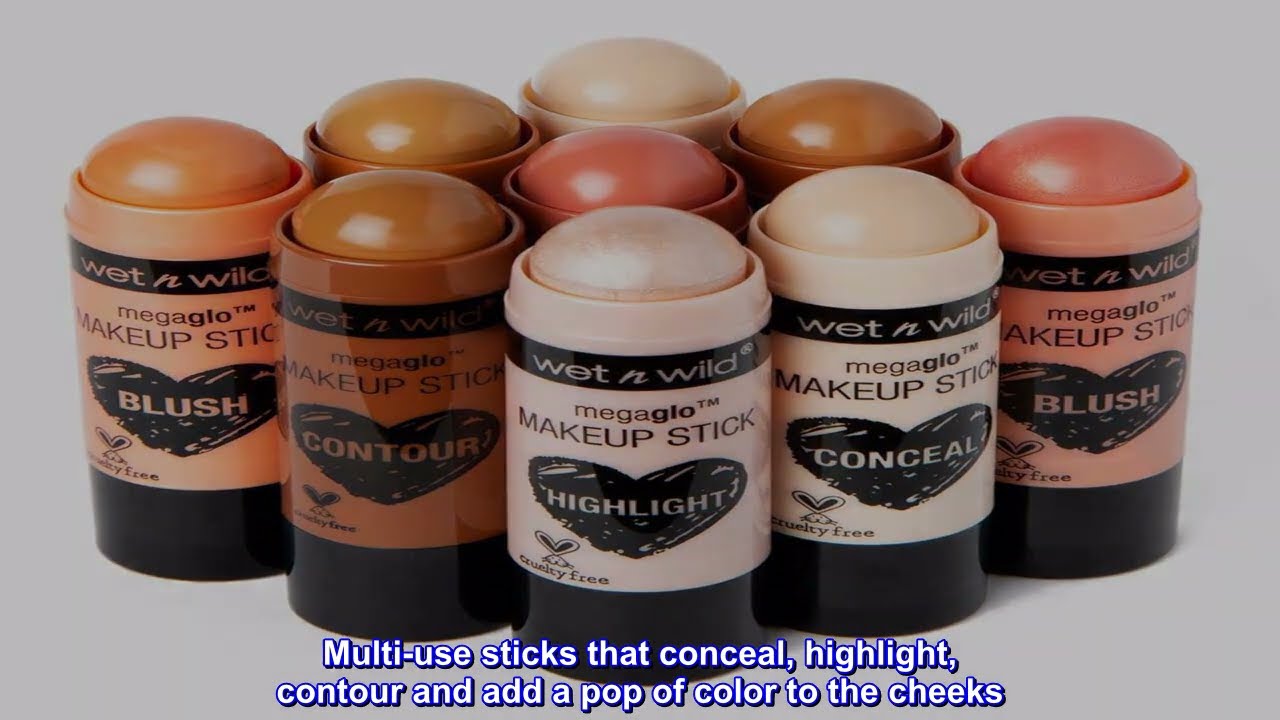This image features nine Wet n Wild Mega Glow Makeup Sticks arranged in a diamond pattern against a white background. Each stick is topped with a rounded cap that resembles roll-on deodorant and color matches the multi-color labels on the canisters. The containers are various shades of pink, orange, brown, and pale skin tones. Each stick is adorned with a black heart that indicates its purpose: blush, contour, highlight, or conceal. The front labels also include the Wet n Wild logo in white font on a black background. At the bottom of the image, there is a caption in white font with a blue border that reads, "Multi-use sticks that conceal, highlight, contour, and add a pop of color to the cheeks." The image emphasizes the convenience and versatility of these cruelty-free makeup sticks, designed for easy application without the need for additional tools.